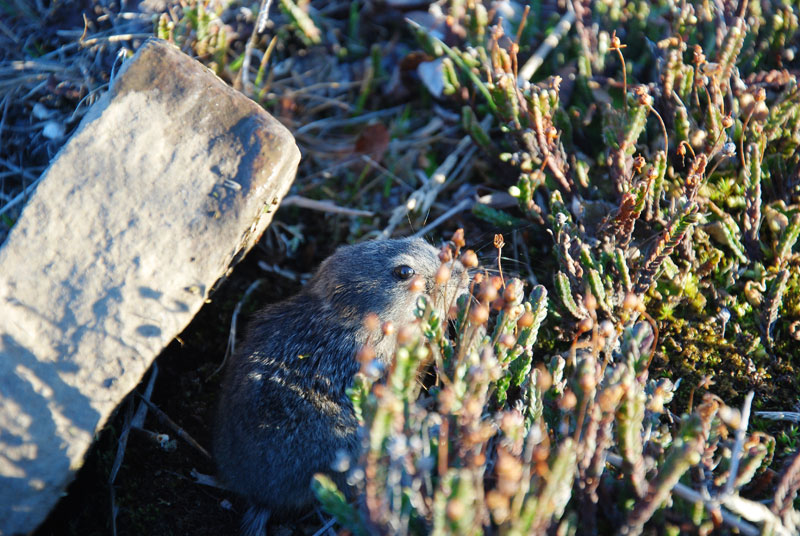This photograph captures a small creature, possibly a ground squirrel or chipmunk, partially hidden behind a patch of mixed green and brown vegetation. The diminutive animal is obscured enough that its full identity is uncertain, but its gray and brown fur, with hints of black, and the glimpses of its eyes and back, suggest it may be a ground squirrel. It appears wary and on alert, perhaps preparing to flee. To its left, a rectangular slab of limestone-like rock juts diagonally from the ground, casting a shadow over the scene. The picture is taken at a low angle, offering a close-up view that emphasizes the ground level details, from the light filtering through the weeds and grasses to the textures of the leaves and stone. The squirrel or chipmunk is centered in the midst of this natural setting, blending into its surroundings, making it an engaging and detailed nature shot.